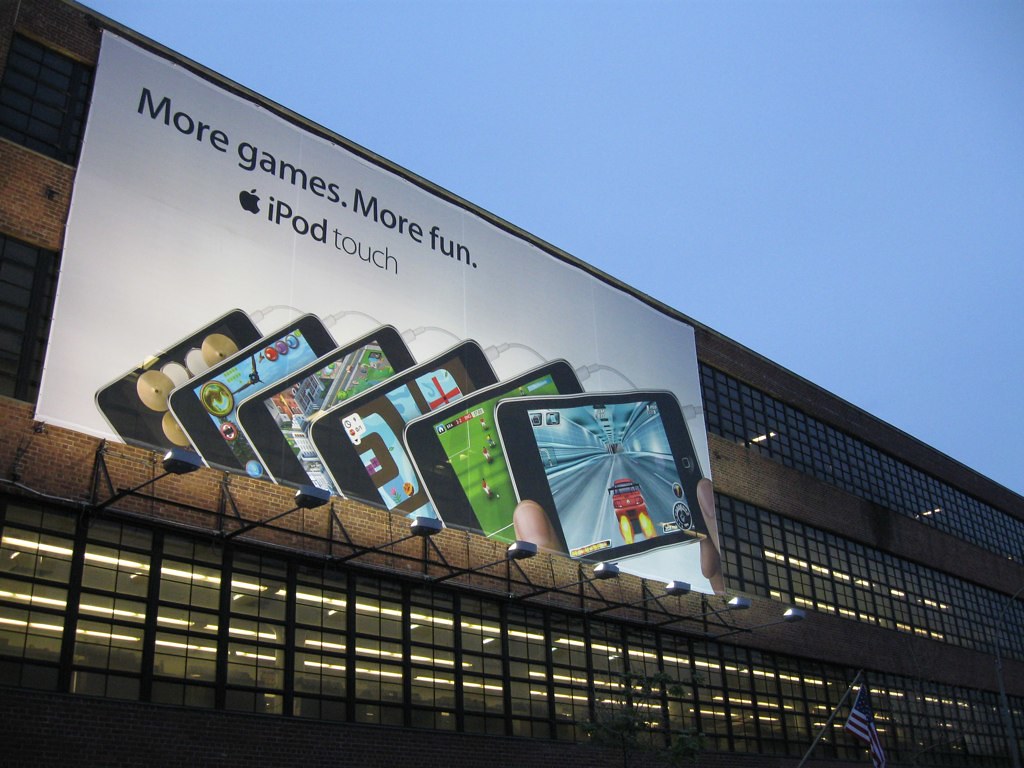This image captures a nighttime cityscape with a prominent three-story building as its focal point. Dominating the side of the building is a large white billboard brightly illuminated by spotlights mounted below. The billboard features the text "more games, more fun, iPad touch" written in bold black letters in the upper left corner. 

Beneath the text, there are six overlapping images of iPads arranged horizontally from left to right, with the foremost iPad fully visible. The foreground iPad, held with visible thumbs, showcases a sleek design, while the partially visible iPads behind it display various colors. 

The building itself has a flat facade and numerous lit windows that suggest an active evening inside. On the bottom right corner of the building, a flag is visible, contributing to the dynamic elements of the scene. The sky above is a deep, rich blue, indicating the late hour, and providing a striking contrast to the illuminated billboard and building below.